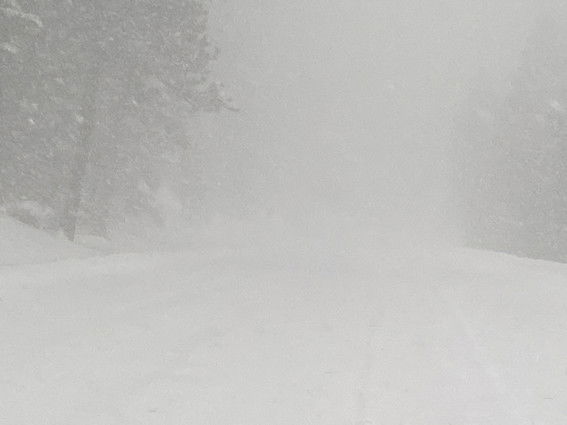This image captures a snowy road engulfed in whiteout conditions, reminiscent of a recent blizzard. The visibility is extremely low due to the dense fog and falling snow, creating a scene that feels like navigating through a thick mist. The road, entirely blanketed in snow, has clearly been plowed, forming embankments of snow on either side. Flanked by large, evergreen trees laden with snow, these trees stretch from the foreground into the blurry distance, their snow-covered branches adding to the wintry ambiance. Small specks of snowflakes continue to fall at an angle, intensifying the scene's frosty atmosphere. The fog extends from the ground up to the treetops, rendering the farther details nearly invisible and emphasizing the harsh weather conditions.